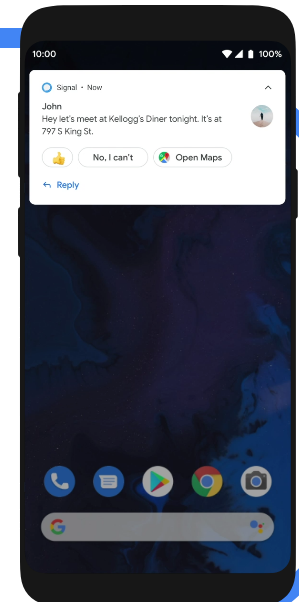A high-resolution screenshot of a smartphone, possibly an iPhone, displaying an open message in the Signal app. The message is from John, suggesting a meet-up at Kellogg's Diner located at 797 South King Street. The recipient has options for responding, including thumbs-up and "No, I can't," with an additional option to open Google Maps to locate the address. The phone is fully charged at 100%, connected to Wi-Fi with full signal strength (four bars), and appears to be logged into a Google account, as indicated by the presence of Google services icons such as Make a Phone Call, Check Messages, Google Play, Google Chrome, and Take a Picture. The home screen background is a dark, satellite-style map with various shades of blue, though its details are somewhat indistinct and primarily black and blue. The overall theme appears to blend technological efficiency with navigational tools.